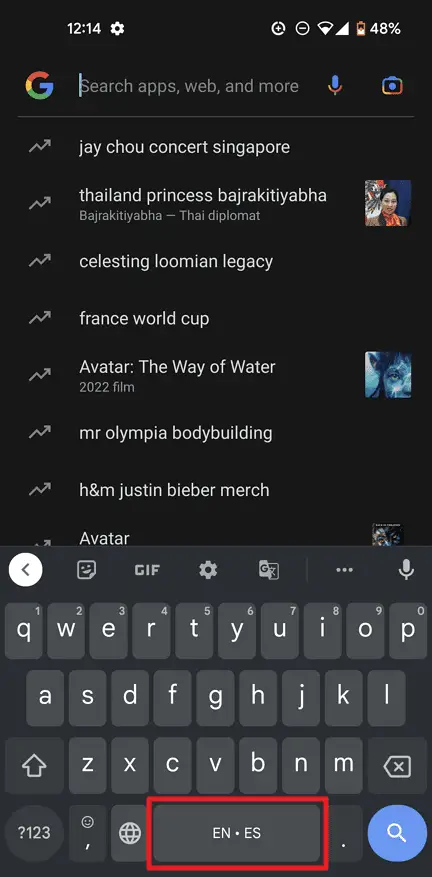A detailed image description of a smartphone screen with a focus on educational purposes: 

The screenshot depicts a smartphone interface showcasing a black background with white text elements. At the top-left corner, the time is displayed as "12:14". Adjacent to it is the settings icon. On the right side of the status bar, the battery indicator shows "48% battery", alongside icons representing active Wi-Fi connection and "Do Not Disturb" mode.

Directly beneath the status bar, a Google search bar features prominently. The "G" logo, adorned in red, yellow, green, and blue, is situated on the left, followed by the text "Search apps, web, and more". A microphone and camera icon are placed to the right of the search bar, indicating options for voice and visual inputs.

Below the search bar, a pop-up keyboard is visible, displaying standard QWERTY keys outlined in red against a black background. In the middle of the keyboard, the space bar is labeled "EN.ES", indicating a dual-language input option between English and Spanish.

There is a post-editing rectangle around the search bar, suggesting the role of the screen in an educational context. This indication is reinforced by the highlighted or annotated elements, as are typical in instructional materials.

The search suggestions or history shown within the search bar include:
1. "Jay Chow Concert Singapore"
2. "Thailand Princess"
3. "BAJRAKITTIYABHA, Thai Diplomat"
4. "Celestial Lumen Legacy" (spelled “Loomian Legacy”)
5. "Finance World Cup"
6. "Avatar: The Way of the Water, 2022 film"

These terms hint at a variety of subject interests, ranging from concerts to royal figures, games, sports, and films.